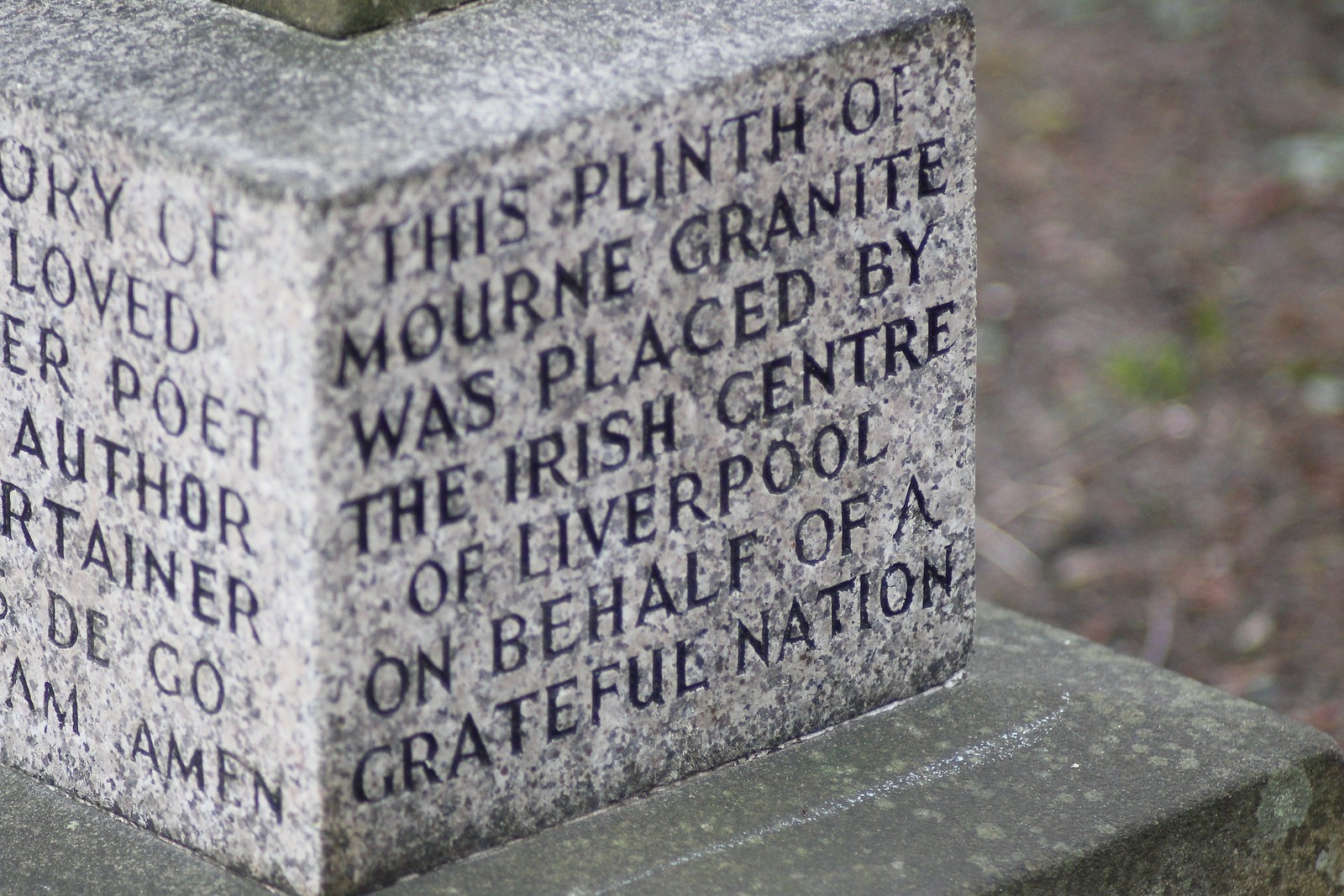This close-up color photograph captures a granite memorial marker outside, glistening from recent rain. The marker, made from light-colored Mourne granite, sits atop a damp, darker cement base. The granite's delicate almost-white hue contrasts starkly with the dark, etched inscription which reads: "This plinth of Mourne granite was placed by the Irish Center of Liverpool on behalf of a grateful nation." The photo is taken at an angle, displaying both the front and partially the left side of the marker, although some letters on the left are obscured, suggesting additional text referring to perhaps a poet or author. Surrounding the memorial, out-of-focus autumn leaves litter the ground, adding a seasonal touch to the scene.